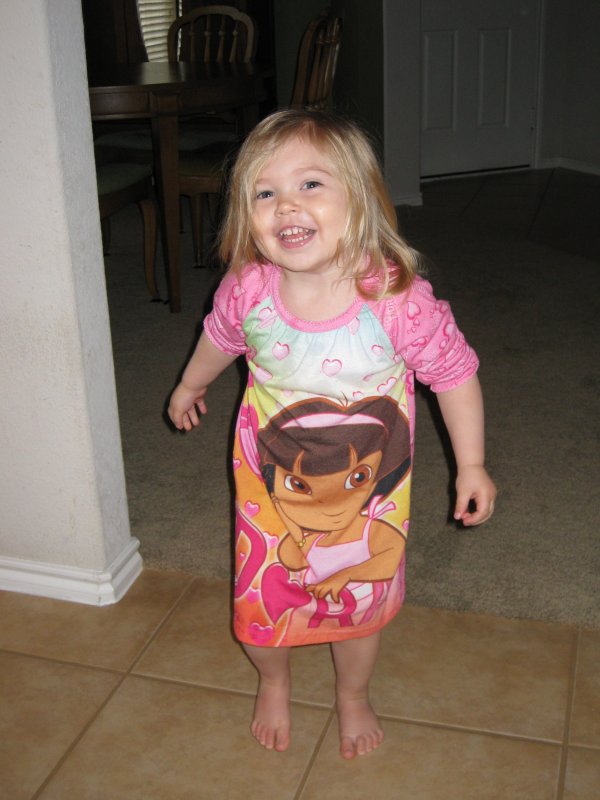In this indoor photograph, a young blonde girl with shoulder-length hair is the central focus. She is smiling brightly at the camera, leaning slightly forward as if to emphasize her cheerful expression. Wearing a nightgown that features a prominent Dora the Explorer design, the bottom part of her attire showcases Dora holding a heart with the name "Dora" written beneath. The top part of the nightgown is adorned with little hearts and is predominantly pink with sleeves bunched up around her elbows.

The setting appears to be a domestic home, suggested by the brown tiled floor the girl is standing on, likely part of the kitchen area. Behind her, a dimly lit, carpeted room is visible, divided by a white wall. A white door is situated in the upper right-hand corner, while a dining table and chairs can be seen towards the upper left-hand corner. The photograph, seemingly taken with a flash, captures the warmth and everyday charm of suburban life.